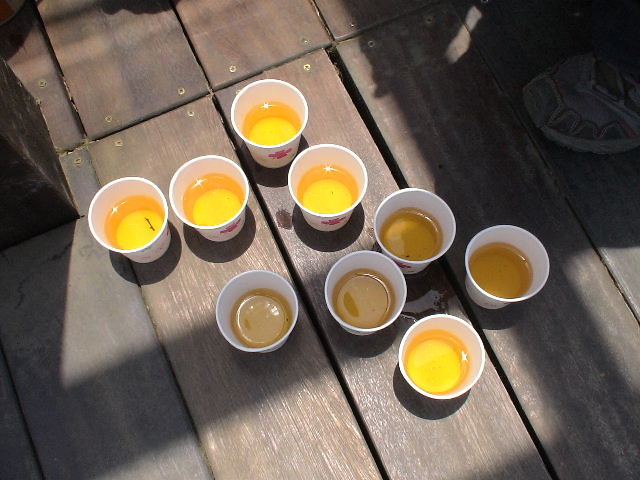This aerial snapshot captures nine white styrofoam cups filled with varying shades of yellow liquid, reminiscent of honey or perhaps different types of juice. The cups prominently display red writing on their sides, though only glimpses can be seen due to the angle. The liquid in five of the cups is a bright, shiny yellow, while the liquid in the remaining four is a deeper, more golden hue. The cups rest on wooden planks, likely part of a deck or porch, showcasing the outdoor setting. The planks are held together by screws, adding an element of rustic charm. Bright sunlight casts pronounced shadows over the scene, including a faint shadow of a sneaker intruding from the top right, hinting at a nearby presence. Overall, the image combines natural light, simple materials, and intriguing liquids to create a visually arresting composition.